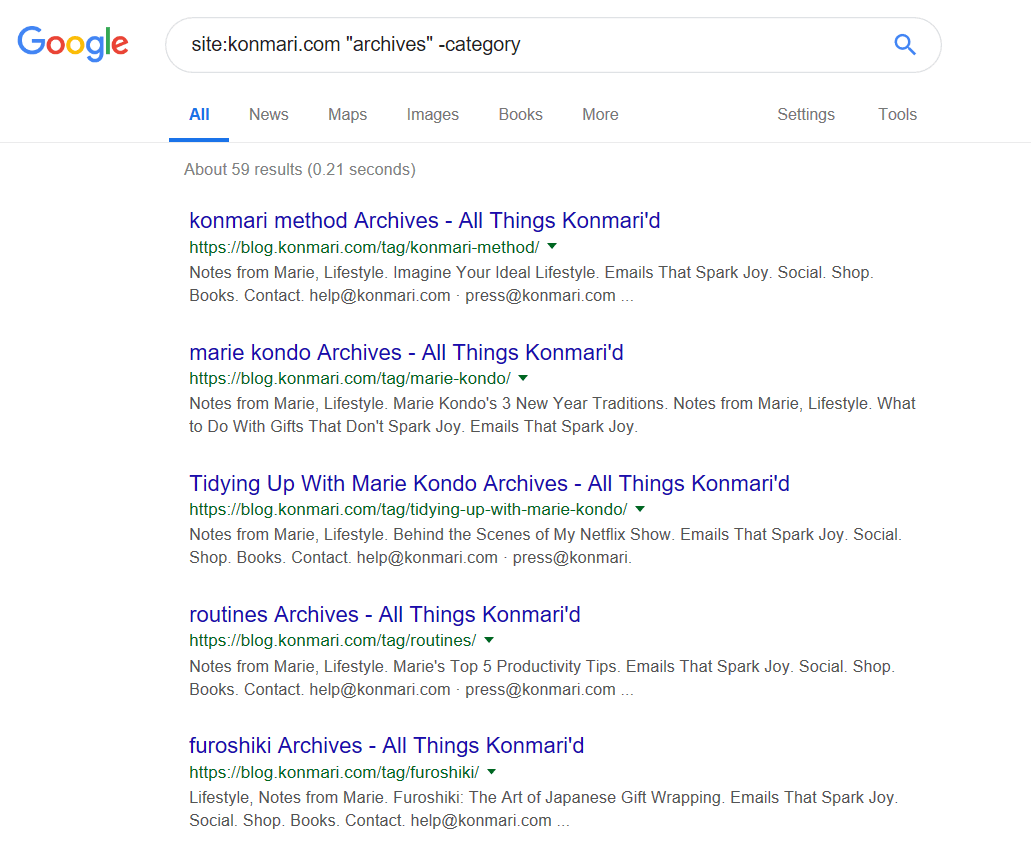Portrait-oriented photo of a Google search screen against a white background, featuring no defined borders. In the top left corner, the colorful Google logo is displayed, with each letter in a different color: a blue capital 'G,' a red 'O,' a yellow 'O,' a blue 'G,' a green 'L,' and a red 'E.' Adjacent to the logo is a long, narrow search bar with the query "site:KonMari.com archives category," accompanied by a blue search icon on the right.

Below the search bar, there are filter options presented in gray text, reading: "All," "News," "Maps," "Images," "Books," and "More," followed by "Settings" and "Tools" on the far right. The "All" filter is highlighted in blue, indicating it is currently selected, with a blue underline for emphasis. A gray border separates the filters from the search results.

The search results section begins with the note in gray text: "About 59 results (0.21 seconds)." The results include multiple blue links, such as "KonMari method archives," "Marie Kondo archives," "Tidying Up with Marie Kondo archives," "Routines archives," and "Furoshiki archives." Beneath each blue link is a green URL and a brief description in black text. The search results suggest an interest in Marie Kondo, a renowned organizing expert, and the user seems to be exploring organizational techniques and routines.